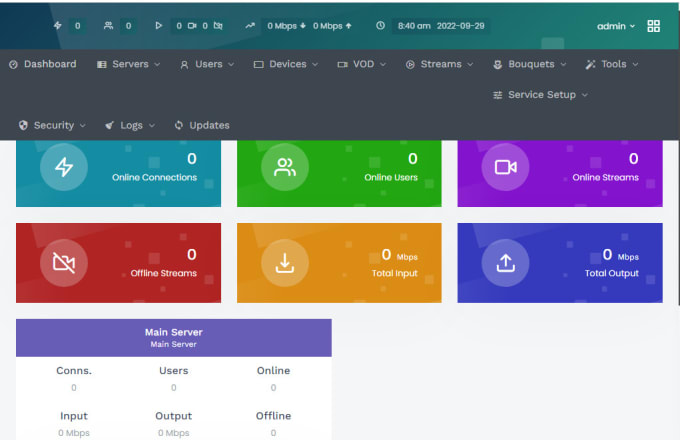This image is a screenshot of a website's dashboard interface. At the top, there is a navigation bar with clickable options, including "Dashboard," "Servers," "Users," "Devices," "Void," "Streams," "Bouquets," "Tools," "Service Setup," "Security," "Logs," and "Updates."

Below the navigation bar, the interface is organized into two rows, each containing three rectangular information panels. 

- In the top row:
  - The first panel is a teal box labeled "Online Connections," indicating a count of zero.
  - The second panel, also teal, is labeled "Online Users," with a zero count.
  - The third panel, showcasing a video camera icon, is labeled "Online Streams," again with a count of zero.

- In the second row:
  - The first panel is labeled "Offline Streams," showing a count of zero.
  - The second panel lists "Total Input," which is also zero.
  - The third panel indicates "Total Output," marked with a zero count.

At the bottom of the interface, there is an additional section dedicated to the "Main Server."